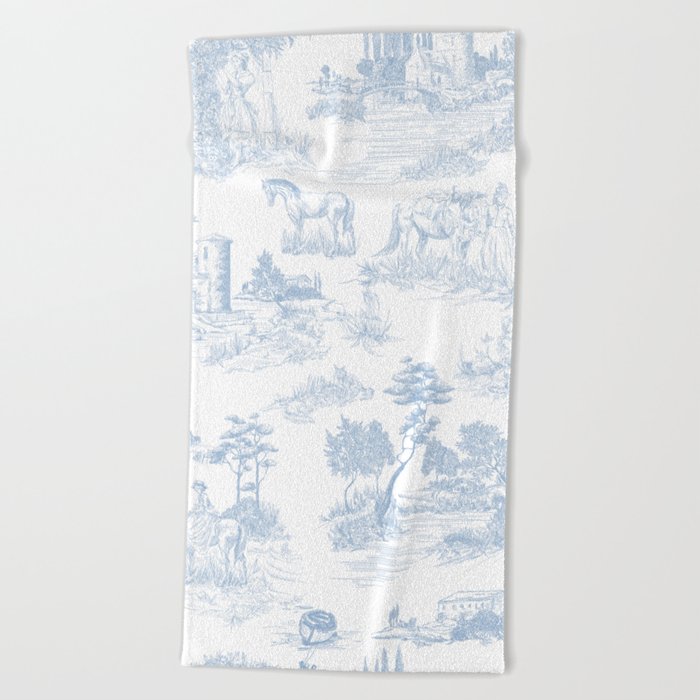The image depicts a piece of toile fabric, possibly a wall tapestry or hand towel, featuring a detailed and intricate pale blue pattern on a white or light grey background. The fabric is rectangular and appears to be a fuzzy, terry cloth material. The toile pattern displays a Victorian-inspired scene with various elements: a stone building resembling a church or monastery with steps and bushes in the middle; a horse standing in a meadow and another horse being led by a woman in Victorian attire; a sketch-like portrayal of various landscapes including a lighthouse situated on an island near water with mountainous and grassy areas in the background; a person on horseback at the bottom left-hand corner, appearing to ride out of the fabric near a lake with a canoe and a small house surrounded by bushes. Additional elements include a long tree with leafy branches, other Victorian-style buildings, and a signature of the artist at the very bottom.